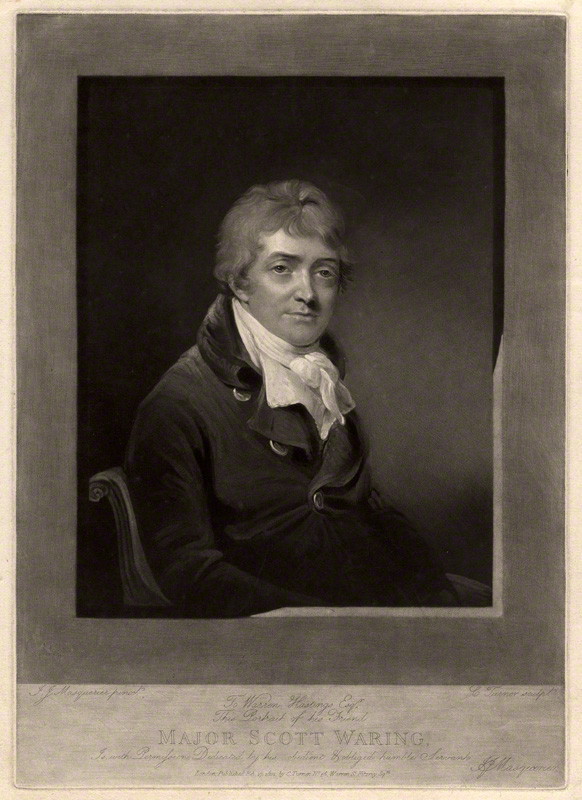The image depicts a black-and-white, old-timey portrait of a middle-aged Caucasian man named Major Scott Waring. The man, who has dark hair of medium length and a long nose, wears a black coat with the top button undone, appearing slightly small for his frame. The coat has dark, long sleeves, and he sports a white scarf around his neck, neatly covering the open part of the jacket. He sits on a carved wooden chair with a distinctive curved back against a gray background. His expression is stoic, gazing off into the distance. The bottom of the image features faint writing with the name "Major Scott Waring" prominently displayed in large print, accompanied by additional cursive text that is difficult to decipher.